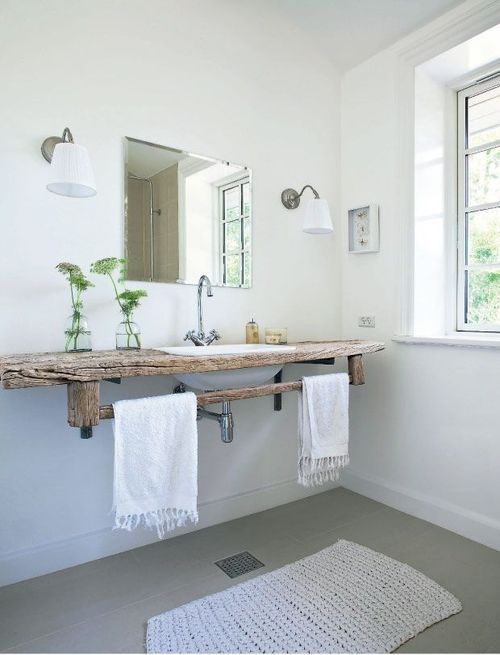In this portrait-oriented, color photograph of a bathroom, we are introduced to a meticulously designed and stylish space, with considerable thought and investment evident in its aesthetics. The bathroom walls are painted a pristine white, complementing the clean and serene ambiance. At the center of the image is a square mirror, reflecting the room's elegance.

The focal point, however, is the washbasin area. The sink itself is a standard white basin flanked by a tall, modern faucet that adds a touch of sophistication. What truly sets this scene apart is the unique counter that anchors the sink. It is crafted from a piece of wood that resembles driftwood, lending a rustic charm with its weathered and character-filled appearance. This plank of wood, reminiscent in size to a small surfboard, is expertly flat and follows the top edge of the basin.

A notable feature of this wooden counter is an extension which seamlessly transitions into a rail-like structure, designed to hold small, white face cloths that are draped elegantly across it. These details collectively create a harmonious blend of modernity and natural elements, making the bathroom both functional and aesthetically pleasing.